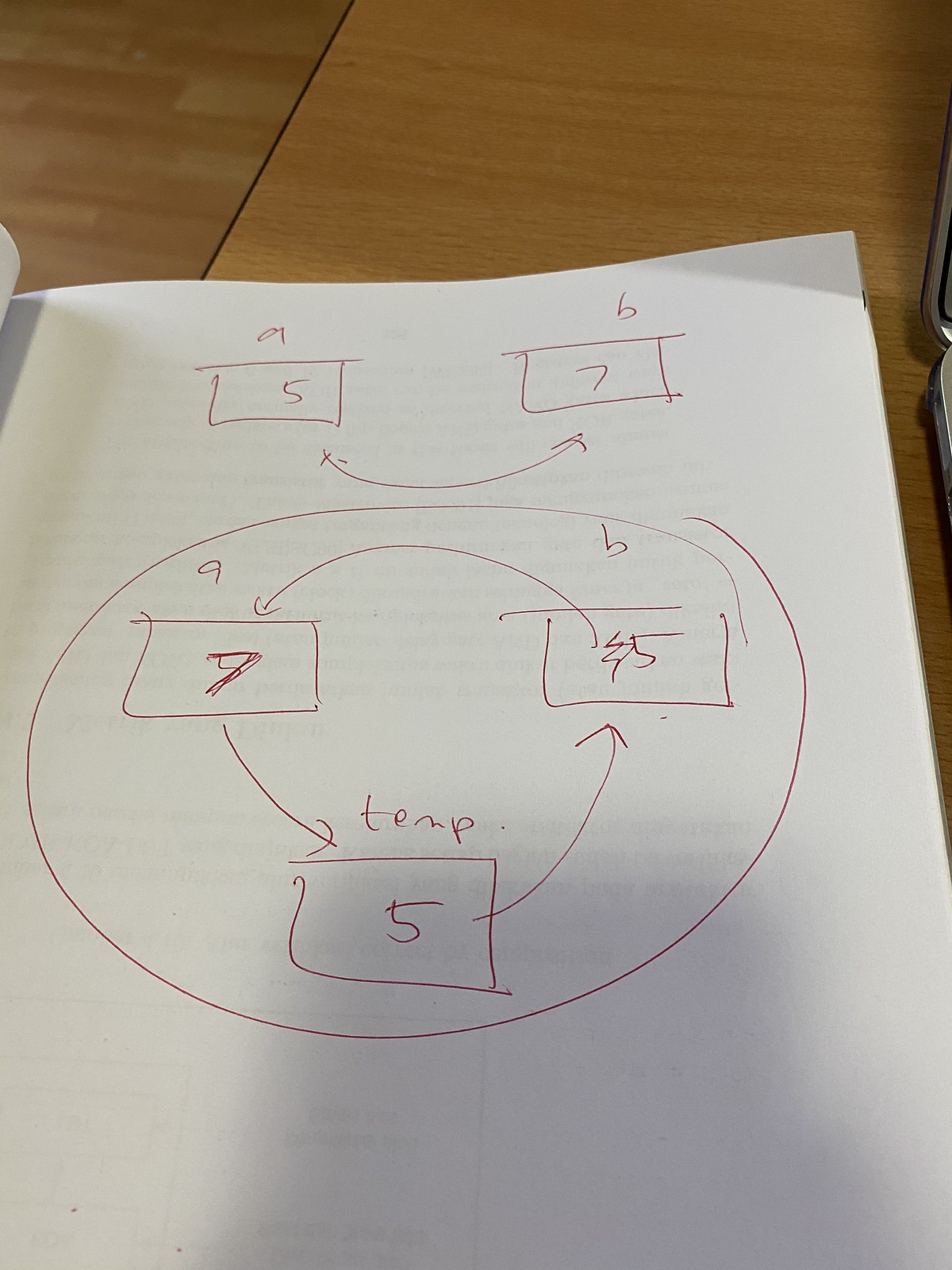This image features a detailed diagram drawn on lined notebook paper. At the top of the diagram, there are two squares, each spaced about an inch apart. The left square contains the number "5" with the letter "A" labeled above it, while the right square contains the number "7" with the letter "B" labeled above it. A curved, bidirectional arrow connects the two squares, positioned below them.

In the center of the image, there is a large circle housing a smaller inner circle. Within this inner circle are three squares arranged in a triangular formation: two at the top and one at the bottom. The left top square contains the number "7," the right top square contains the number "5," and the bottom square contains the number "5" as well. The word "temp" is written just above the bottom square. All three squares are interconnected with arrows featuring arrowheads, indicating a flow or relationship between them.